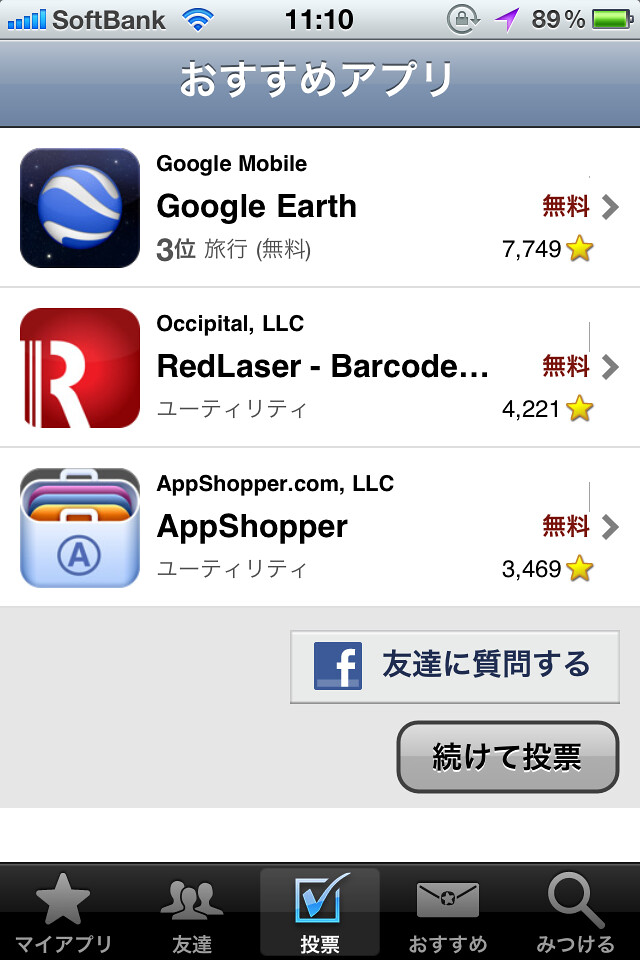The image is a color screenshot of a smartphone in portrait orientation, displaying what appears to be an iPhone interface in Japanese. The top part of the screen shows the SoftBank carrier information, full signal bars, Wi-Fi status, and an 89% battery level, along with a purple icon resembling a Star Trek symbol. Below this, a light gray gradient header features several Japanese characters in white.

The main content consists of app listings presented in white horizontal rectangles, each with an icon to the left. The first app listed is Google Earth, sporting a black icon with a blue and white globe, labeled "Google Mobile" above it and accompanied by a star rating and Japanese text in dark red to the right. The second app is RedLaser, known for barcode scanning, and the third is AppShopper, both following the same format as Google Earth.

Further down, the Facebook logo appears, flanked by Japanese typography, and another button below it with more Japanese text. At the screen's bottom, a black horizontal bar contains five gray navigational icons: a star, a people icon, a checkmark, an envelope, and a magnifying glass. The detailed layout and Japanese language suggest an app-related interface tailored for users familiar with both the language and the featured applications.